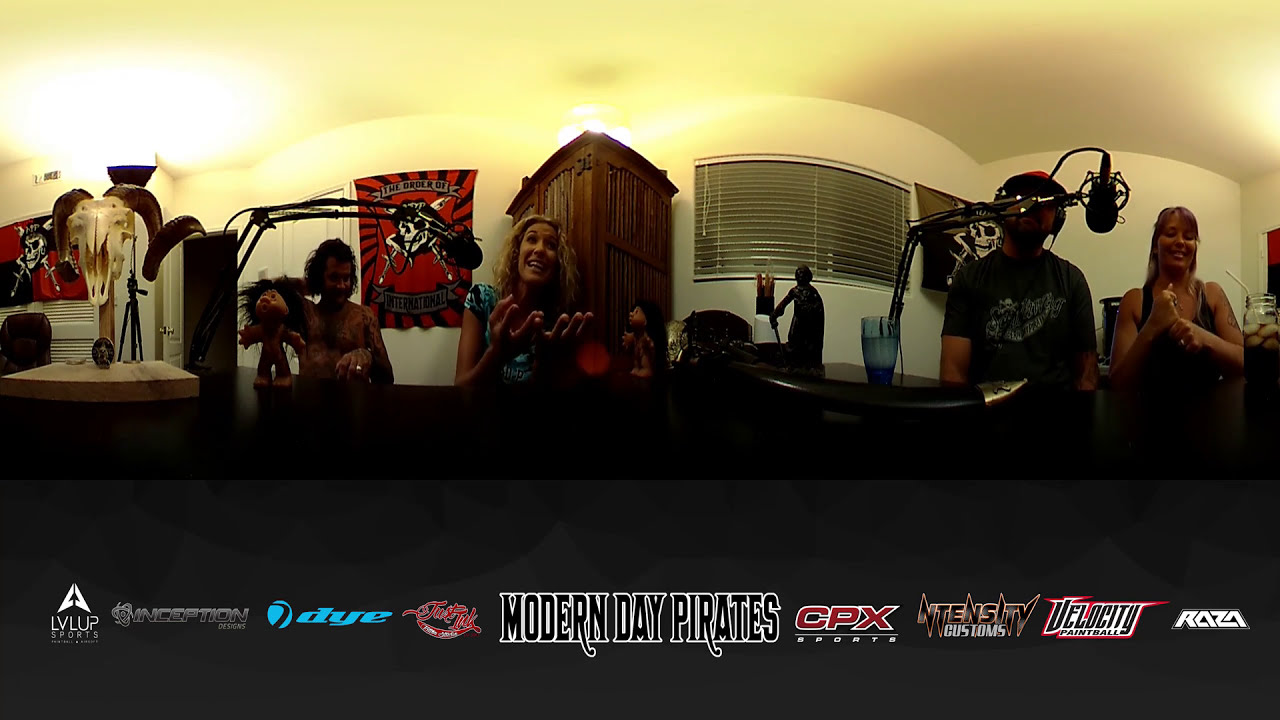The image is a 360-degree panoramic photo of a recording studio with plain white walls adorned with a few black, red, and white posters, including some featuring skulls. There is a collection of troll dolls adding a quirky touch to the space. The studio features mechanical arm microphones extended out towards the individuals present. 

Starting from the left, there's a shirtless man with long black curly hair and tattoos, scratching the back of his head. Next to him, a cheerful blonde woman with curly hair is animatedly speaking into a microphone, her hands raised mid-gesture. Further to the right, a man wearing a black t-shirt and a baseball cap has headphones on and is positioned in front of another microphone. To the far right, another woman with dark hair and bangs, dressed in a black tank top, holds an iced drink.

At the bottom of the panorama, various slogans and brand names are featured, including "LVLUP," "Inception," "DYE," "Modern Day Pirates," "CPX Sports," "Intensity Customs," "Velocity Paintball," and "RAZA," contributing to the vibrant and energetic atmosphere of the studio. Overall, the individuals appear to be in their 30s, engaged and interacting within the lively setting of the recording studio.